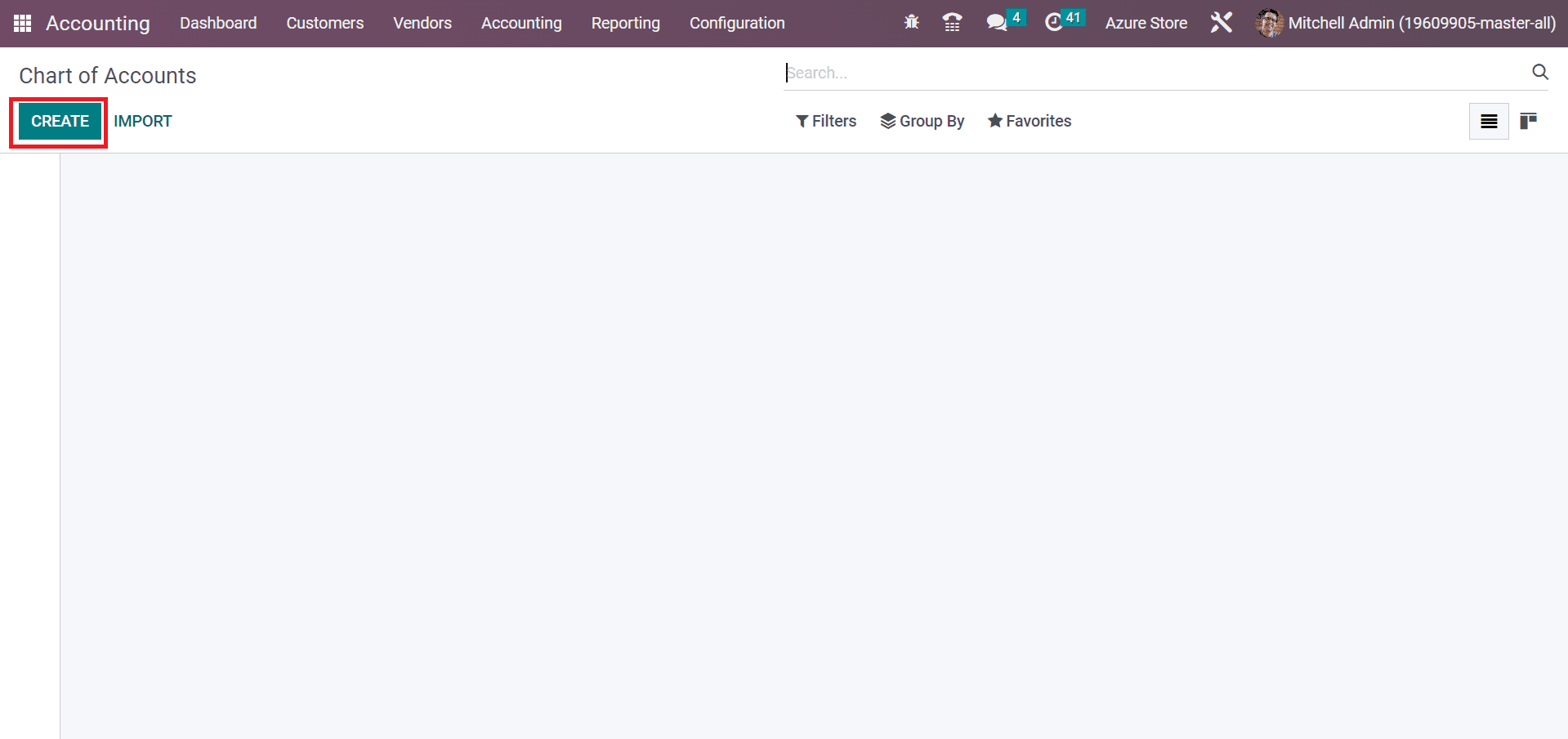This image is a screenshot of a webpage from a website called Azure Store, which appears to be a comprehensive accounting software. The top menu bar includes options for navigation, listed from left to right: Accounting, Dashboard, Customers, Vendors, Accounting, Reporting, and Configuration. Additionally, the bar features several icons, including a message icon, a clock icon, the Azure Store logo, a settings icon, and the account name, Mitchell Admin, indicating the current logged-in user.

The main section of the page is labeled "Chart of Accounts," which suggests this is a tool for financial data organization. Prominently highlighted in red is a 'Create' button, likely intended to guide users towards initiating a new task or entry. A search bar and various functional tabs—filters, group by, and favorites—are situated below the title, designed to help users manage and sort their data efficiently.

The remainder of the page below these tools is dominated by a large, blank gray box, indicating that there are no current entries or data displayed. The simplistic and uncluttered layout implies that this screenshot is either from a user just getting started or from a moment when no specific accounting data has been entered or loaded yet.